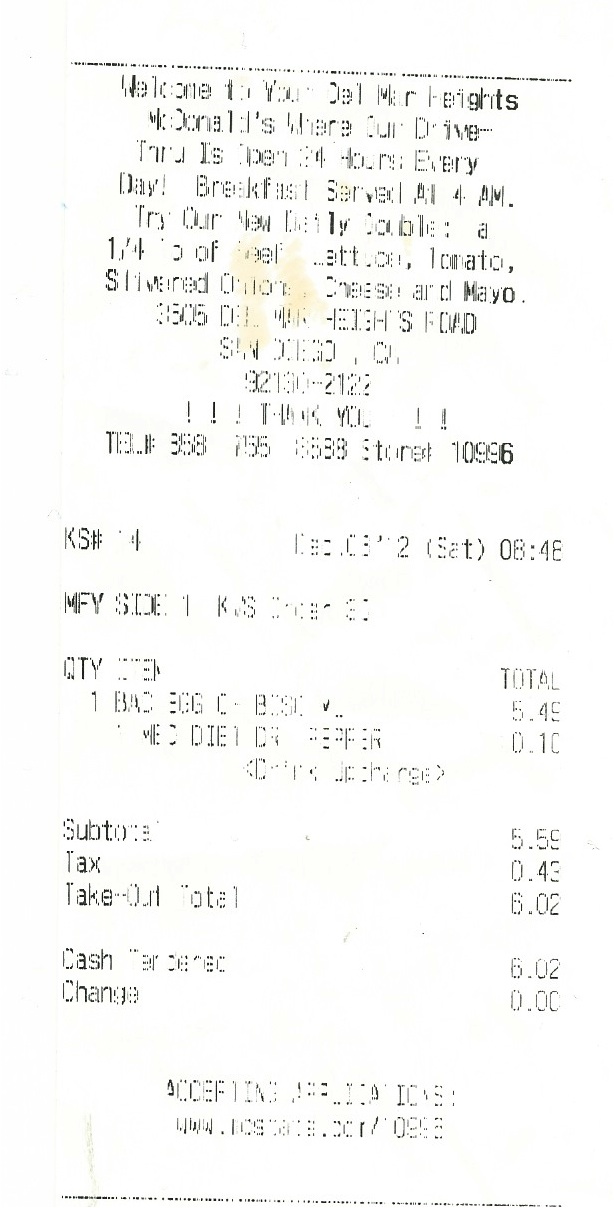This image captures a blurry and slightly stained scanned receipt from a McDonald's drive-thru at Del Mar Heights. The receipt notes that the drive-thru is open 24 hours daily, with breakfast starting at 4 AM. The itemized purchase details include a bacon, egg, and cheese biscuit and a Diet Dr. Pepper, totaling $6.02 with tax, from an initial subtotal of $5.59. The transaction occurred on Saturday, December 8th. Despite the low-quality scan, the receipt also features a promotional note about a new daily menu item with beef, tomato, onion, cheese, and mayo, and a thank-you message along with a blurred-out address.